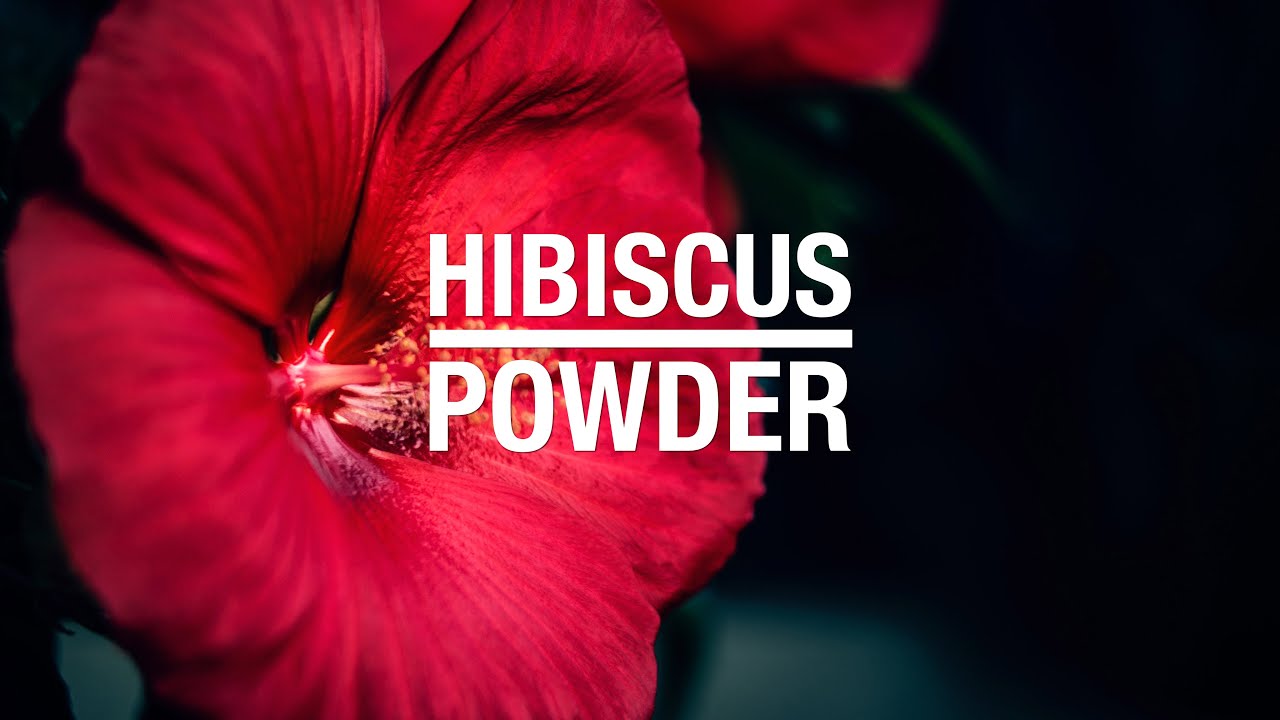The photograph captures a vivid red hibiscus flower against a dark background, predominantly black with subtle hints of gray at the bottom. The flower, positioned on the left half of the image, showcases rich, grooved petals with bright yellow stamen and pistils prominently poking out from the center, giving it a striking three-dimensional appearance. Superimposed in the exact center of the photograph are the words "HIBISCUS POWDER" in capital white letters, with "HIBISCUS" on top and "POWDER" below, separated by a thick line. This text creates a perfect rectangle, standing out clearly against the vibrant red flower and the dark backdrop.